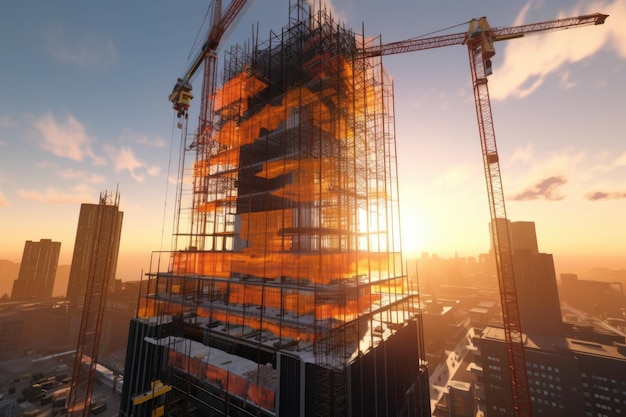This color photograph captures an impressive cityscape at either sunrise or sunset, showing a skyscraper under construction. The scene is dominated by the partially completed high-rise, which has scaffolding all around it and is flanked by two large red cranes positioned on either side. The building’s lower section appears more complete, featuring black windows, whereas the upper part remains a skeletal structure of metal beams and iron rods, reflecting a striking orange hue due to the sunlight filtering through. The bright sun, situated just over the horizon at the center of the image, bathes the entire sky in a blend of golden, pink, purple, and blue tones, casting a romantic and somewhat surreal ambiance over the scene. Surrounding the main skyscraper are several other tall buildings, though none reach its impressive height, amplifying the vertical dominance of the structure in progress. The clear sky, dotted with a few puffy white clouds, enhances the crisp, almost exaggeratedly clean appearance of the photo, leading to some speculation about it being a hyper-realistic illustration or CGI. The image exudes a vibrant yet hazy quality, with the sun’s position and the reflecting glass of the skyscraper giving an impression of the building being almost on fire. The overall atmosphere is one of dynamic urban growth and architectural ambition, set against a serene and richly colored sky.